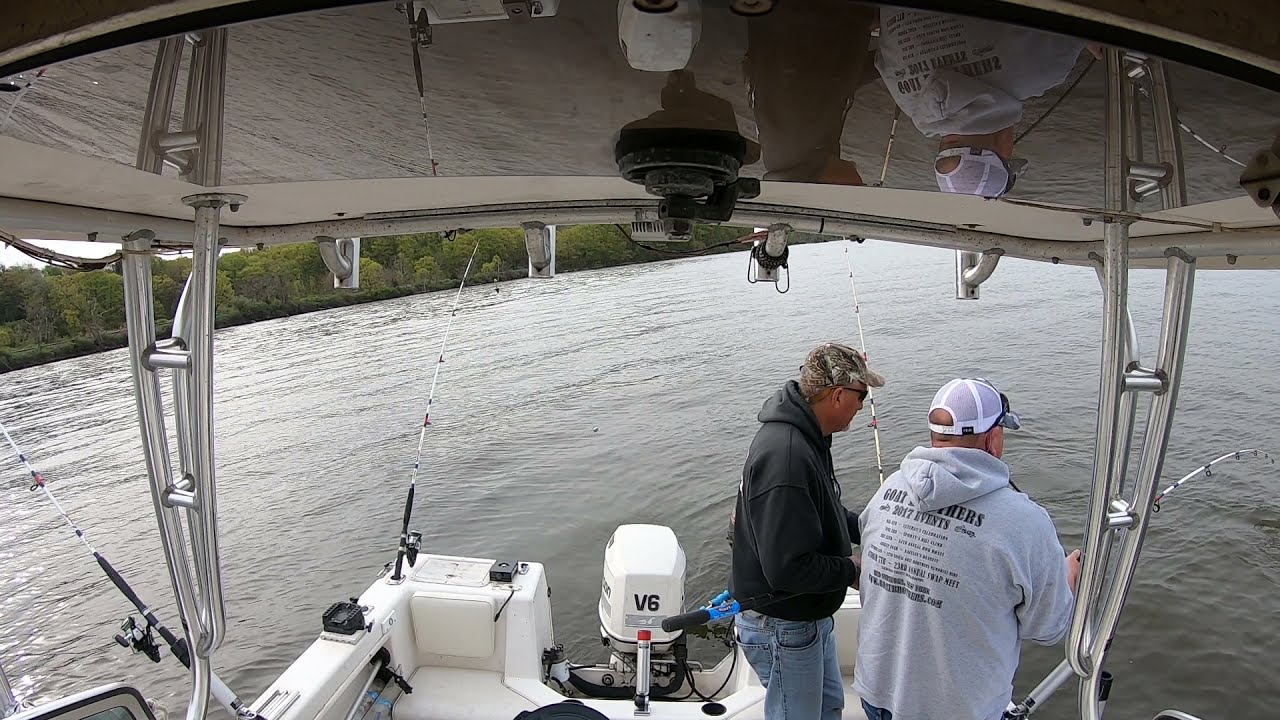In this image, two middle-aged men are standing on the back of a white fiberglass riverboat, equipped for a fishing expedition. The boat, fitted with a V6 outboard engine, is positioned on a murky greenish-brown river, encircled by lush vegetation and possibly marshland. Both men, with their backs to the camera, are engrossed in their fishing endeavor. The man on the right, wearing a white mesh baseball cap and a gray hoodie with "Goat Outfitters 2017 events" on it, holds a fishing rod, appearing to either reel in or maintain his catch. To his left, the second man, dressed in a black hoodie, blue jeans, a camouflage baseball hat, and sunglasses, seems to be either assisting or advising him. In addition to the rods each man is holding, there are two unattended fishing rods on the left side of the boat, seemingly set in their holders awaiting a bite. Ahead of them, the tranquil water reflects their figures, while the boat's top provides some shade. The serene scene captures a moment of recreational fishing, set against the backdrop of verdant riverbanks.